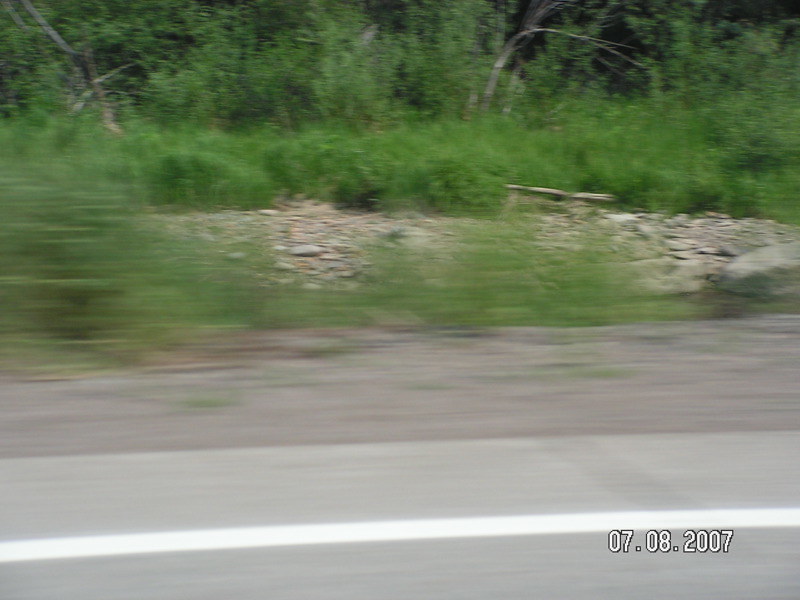This color photograph, slightly blurry and out of focus, appears to have been taken from a moving car, possibly by someone seated in the backseat. The motion blur suggests the car was in transit when the photo was captured. 

At the very bottom of the image, we can see the edge of the gray asphalt road marked by a white line. Just beyond this, the shoulder of the road consists of sandy or dirt terrain. The next visible layer includes an area scattered with larger stones, suggesting a rough, untended ground. 

Further back, a dense growth of wild weeds and bushes dominates the scene, leading into a thick forest that fills the upper portion of the photograph. 

In the bottom right-hand corner, the date “07.08.2007” is visible, indicating when the photograph was taken.